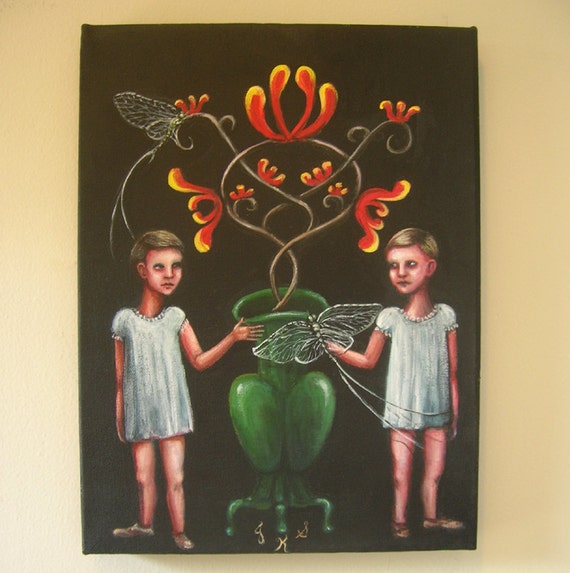The painting, likely rendered on a black canvas, is affixed to a beige wall. It presents two young girls positioned on either side, mirroring each other in a vertical orientation. Both girls have short dirty blonde hair and are dressed in white, short nightgown-like dresses that fall to their hips. They each wear brown shoes and extend their hands towards the center of the composition. Dominating the central space between the girls is a tall green vase with three supportive legs. Rising from the vase is an intricate, twisted brown branch adorned with vibrant, fiery-colored flowers resembling flames, featuring hues of orange and yellow. Two dragonfly-like insects with semi-transparent wings are also present: one near the top left flower and one that the girl on the right seems to be grasping. Additionally, the canvas bears a signature at the bottom, possibly reading "GXS" in yellow. The overall scene is set against a stark black background, creating a strong visual contrast with the vivid elements in the painting.